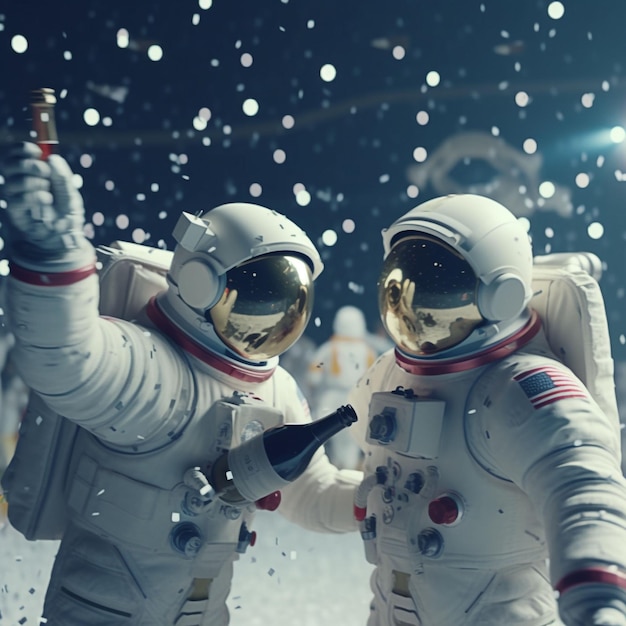The image portrays a close-up of two astronauts dressed in white spacesuits adorned with red borders around their necks, wrists, and numerous buttons on the front. Each astronaut has an American flag patch prominently displayed on their left shoulder. The astronaut on the left is holding a wine glass with their right hand and has a wine bottle strapped to their chest, while the astronaut on the right holds a beer. Both astronauts appear to be celebrating amidst a flurry of confetti, which fills the air with a festive atmosphere. The image, tinged with a yellow hue, hints at a staged or artistic setup, possibly involving toy astronaut figures. In the background, a third, blurry astronaut figure is barely visible, adding depth to the scene. This vividly detailed portrayal encapsulates a moment of joyous celebration, complete with vivid confetti and festive props, set against the intriguing backdrop of space adventure.